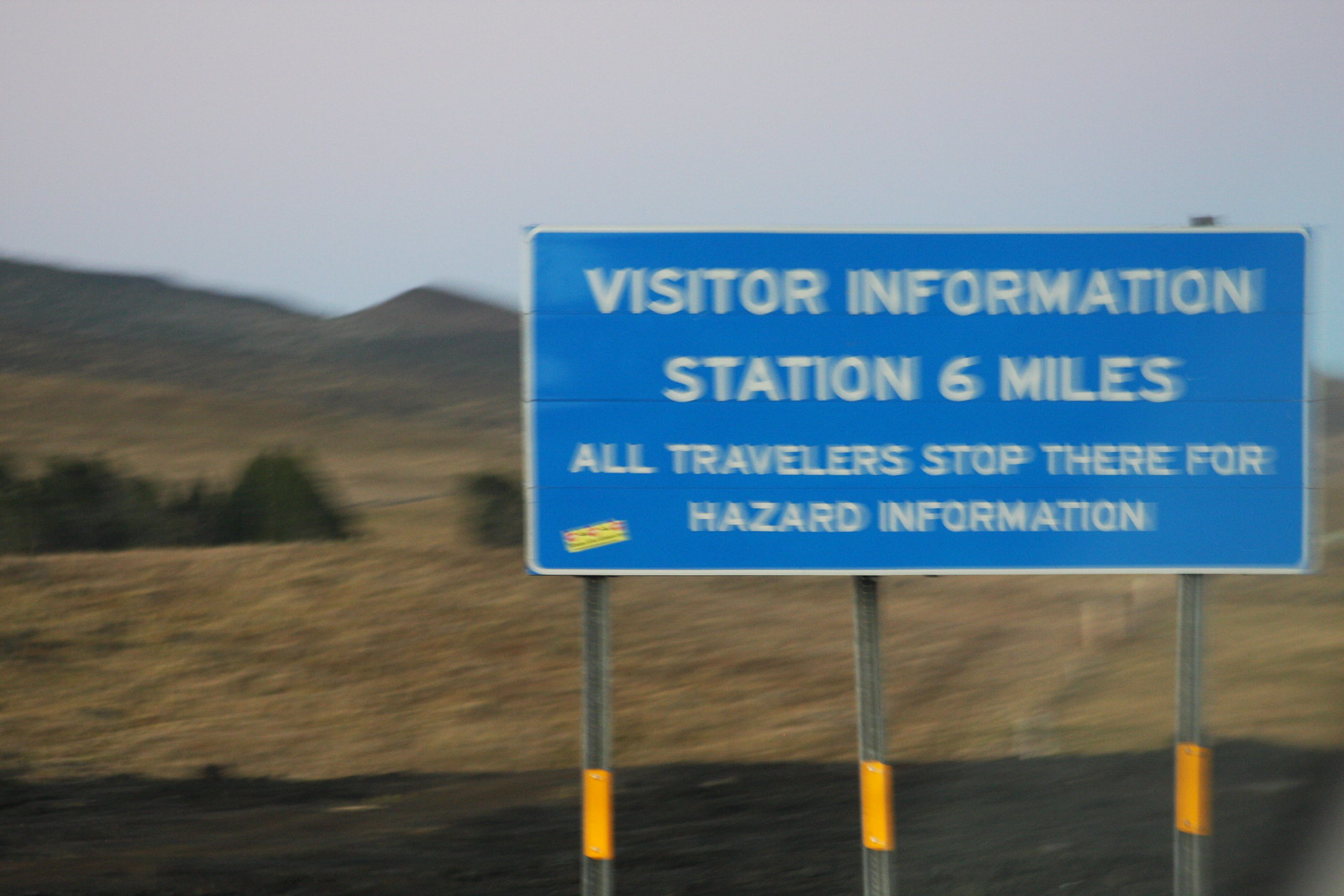The slightly blurred photograph captures a roadside scene taken from a moving car, focusing on a blue informational road sign typical in the United States. The sign, with white lettering, states "Visitor Information Station, 6 miles. All travelers stop there for hazard information." It is supported by three steel poles, with the middle one featuring a yellow reflector for high visibility at night. A yellow sticker is also visible in the bottom left corner of the sign. The landscape behind the sign is hilly and arid, with sparse greenery consisting of some scrub and shrubs scattered nearby. The ground is predominantly brown, suggesting a desert-like environment, while the distant hills appear sloped and brownish. The sky above is pale, with diffuse white clouds giving it an almost white appearance. The photograph also shows a roadway in the foreground, enhancing the sense of a typical roadside setting.